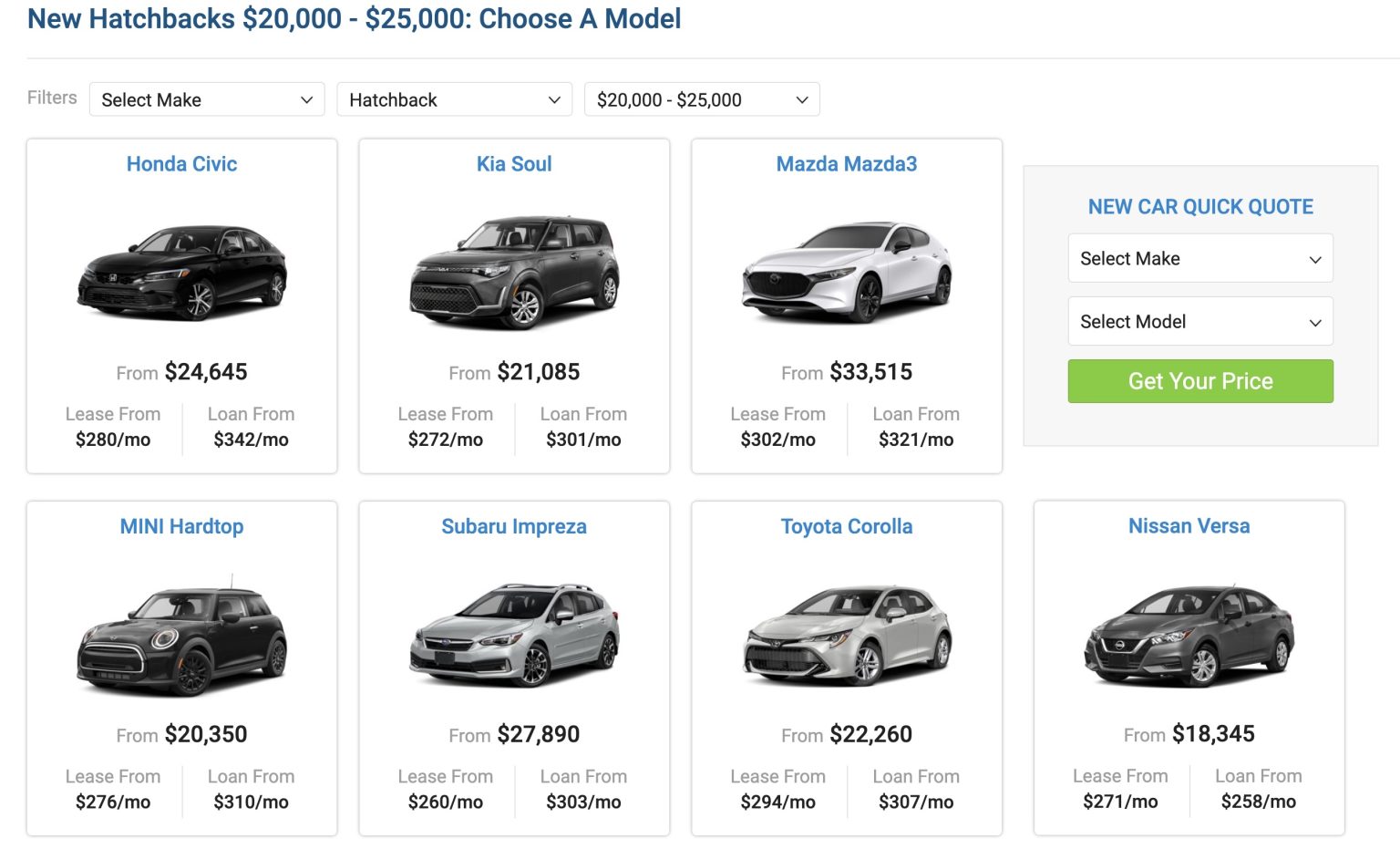The image depicts a segment of a website featuring new hatchbacks priced between $20,000 and $25,000. In the top left corner, a greyish-blue heading reads "New Hatchbacks $20,000 to $25,000 - Choose a Model." Directly beneath the heading, a fine grey line spans the width of the screen, delineating the header from the content below.

Below this line, there are several filter dropdown options designed to help users refine their search. The first filter allows the selection of a specific car make, while the second filter narrows down the car style, such as hatchback. The third filter sets the price range, showing a default value between $20,000 to $25,000.

Under the filters, a series of white tiles display various car models available within the specified price range. Each tile features an image of the car, the car's name in blue text, and the starting price. The tiles also provide information on monthly lease costs and loan estimates. From left to right, the models displayed include:
- Honda Civic from $24,645
- Kia Soul from $21,085
- Mazda Mazda3 from $33,515
- Mini Hardtop from $20,350
- Subaru Impreza from $27,890
- Toyota Corolla from $22,260
- Nissan Versa from $18,345

In the top right corner of the screen, above the Nissan Versa tile, there is a "Quick Quote" section. This feature allows users to select a make and model and receive a price by clicking on a prominent green button.